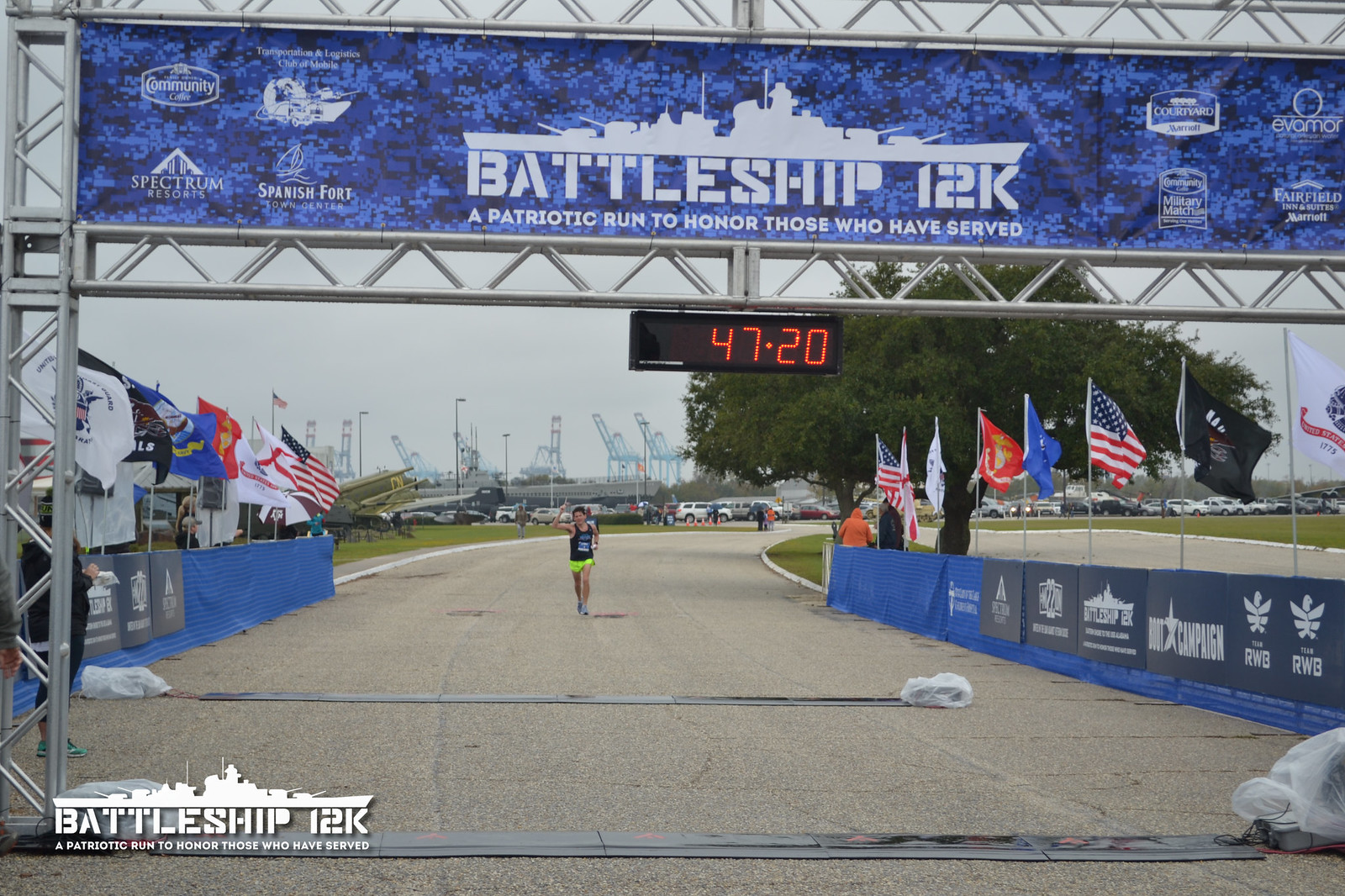The image captures a runner approaching the finish line of the Battleship 12K, a patriotic race to honor those who have served. The finish line is prominently marked by a large metal frame with a blue banner that reads "Battleship 12K, a patriotic run to honor those who have served" in white text. The runner, wearing a blue tank top and neon green shorts, is approximately 25 yards away from the finish line, running on a gray concrete road course. The day is overcast, suggesting a summer event given the light athletic gear worn by the participant.

Flanking the course are blue banners and a collection of flags, including American flags and various military and state flags. The background features city skyscrapers, a parking lot, and what seems to be military jets in the distance. A digital clock above the finish line displays the time as 47 minutes and 20 seconds. Despite the overcast sky, the scene is vibrant with patriotic elements and the clear structure of an organized race.